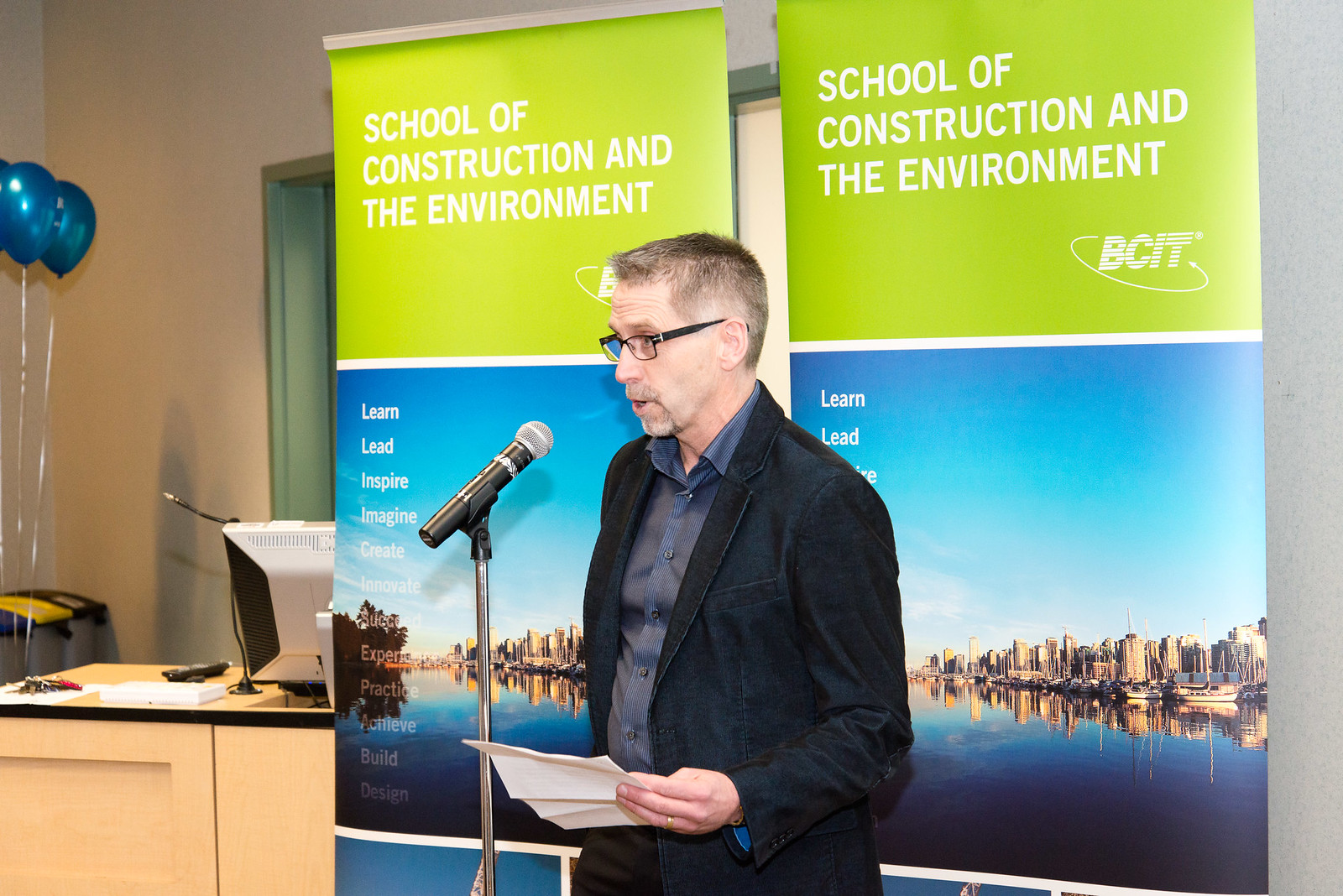In the image, a distinguished man with gray hair stands at a microphone on a stand, addressing an audience. Dressed in a blue suit paired with a blue button-down shirt, he holds a piece of paper in his left hand, his palm facing up. He wears black glasses that add to his scholarly appearance. Behind him, two vibrant posters prominently display the text "School of Construction and the Environment" and "BCIT" in white on a green background. The posters also feature inspirational words like "Learn, Lead, Inspire, Imagine," with additional phrases such as "Build" and "Design" towards the bottom. The backdrop of the poster includes an image of a serene lake encircling a cityscape, with a detailed skyline. To the left of the speaker, two balloons add a touch of festivity to the room, and a desk with a brown top is partially visible. The setting appears to be a formal event or seminar, contributing to the professional atmosphere of the scene.